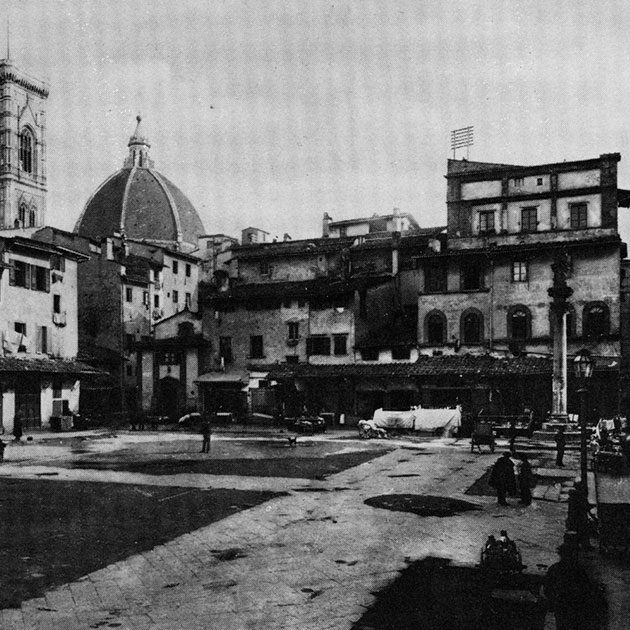This black and white photograph depicts an expansive town square, possibly in Asia or India, characterized by a mix of architectural styles. Dominating the background on the left is a prominent building with a domed roof, featuring supporting arches and culminating in a triangular peak. Adjacent to this dome, a sizable tower with an arched window and oblong windows stands imposingly. The building directly ahead showcases several second-story arched doorways and a square window. To the right, sidewalks and walkways, made of brick and concrete, are populated by various people, with a noticeable cluster near the right side and some small figures on a bench. In front of the background buildings, there is a white oil truck visible. Overall, the scene is tranquil under a clear, unobstructed sky, captured from a distance in slightly lower resolution.